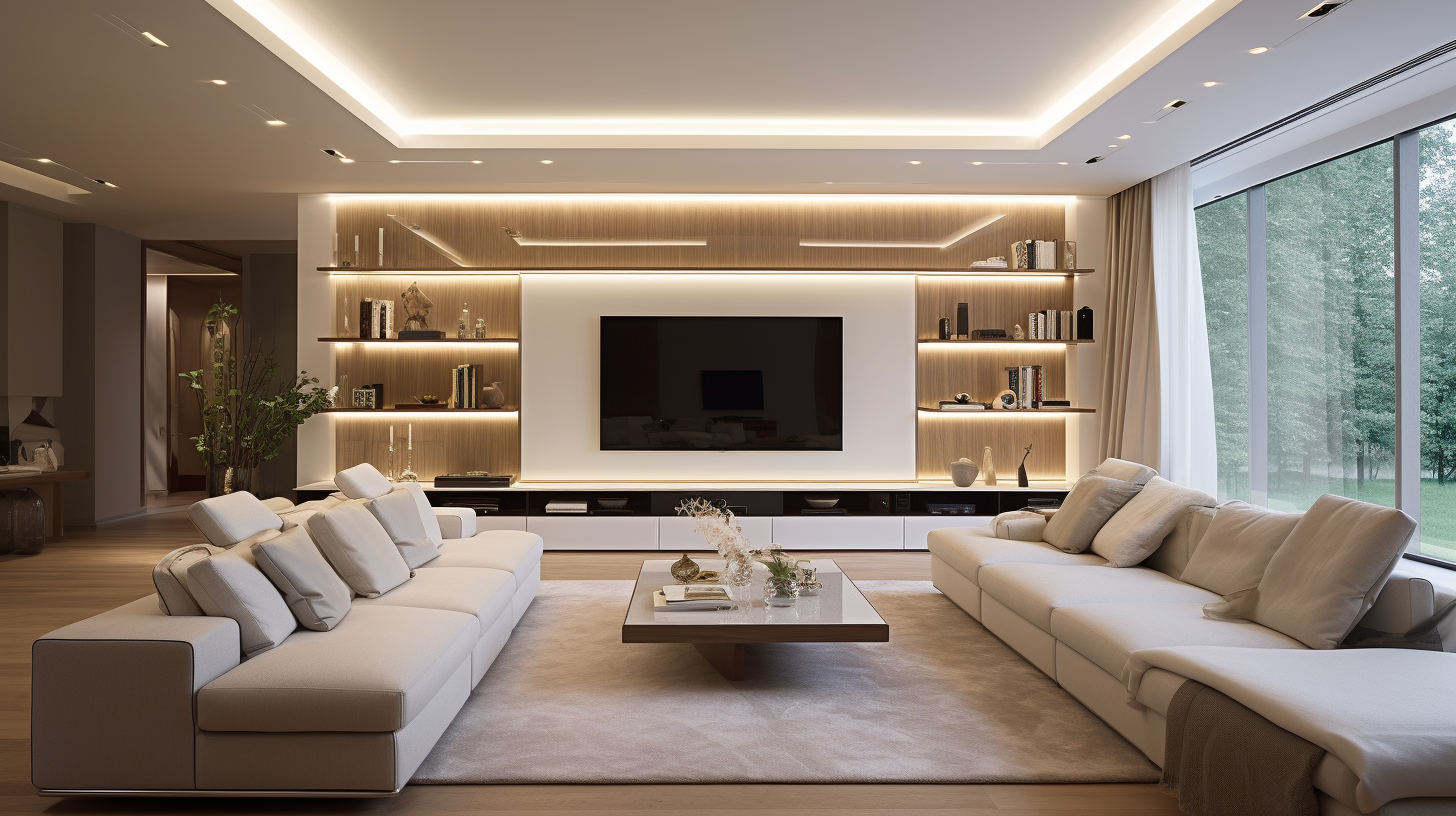This is a professional photograph of a spacious, modern luxury living room taken in landscape orientation, ideal for use in a blog, magazine, or website dedicated to architecture or home décor. The living room features a rich brown wooden floor and a white recessed ceiling with elegant built-in lighting. Dominating the room is a large flat-screen TV mounted on a light wooden wall with LED-lit shelves surrounding it, displaying a variety of books, trinkets, and decorations. 

In the center, a low, modern coffee table with wooden sides and a white top sits on a light gray plush rug. The table is adorned with a small flower arrangement, a wire sculpture, and some magazines. Two off-white couches, seating three to four people each, face each other across the table, both accented with multiple pillows for added comfort. 

To the right, a full wall of glass provides a view of pine trees outside, framed by tan and white curtains on a modern curtain stand. A large potted plant adds a touch of greenery to the left side of the room, enhancing the neutral color palette of black, white, gray, tan, and green. The room is well-lit, with natural light pouring in from the window and additional ambient lighting from the ceiling and shelves, creating a bright and inviting atmosphere.